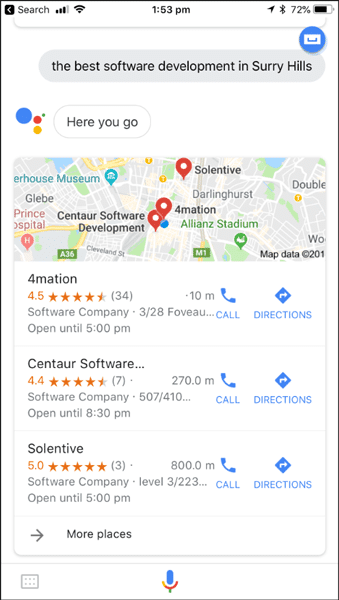This image is a mobile screenshot of a search results page, likely from a search engine resembling Google due to its color scheme, though it lacks the Google logo. The search query displayed in the search box reads "the best software development in Surrey Hills." Below the search bar, there's a text response saying "Here you go," followed by a map featuring several marked locations.

Highlighted business listings include:
1. **Formation** - Features detailed information including address, distance, and a 4.5-star rating, along with buttons to get directions or initiate a call.
2. **Centaur Software Development** - Shows similar details and sports a 4.4-star rating.
3. **Selentive** - This business stands out with a perfect 5.0-star rating, as well as address and navigation options.

At the bottom of the screen, there is a microphone icon, suggesting voice search functionality. The map and listings provide comprehensive contact options, including addresses, distance measurements, and direct links for calling each business.